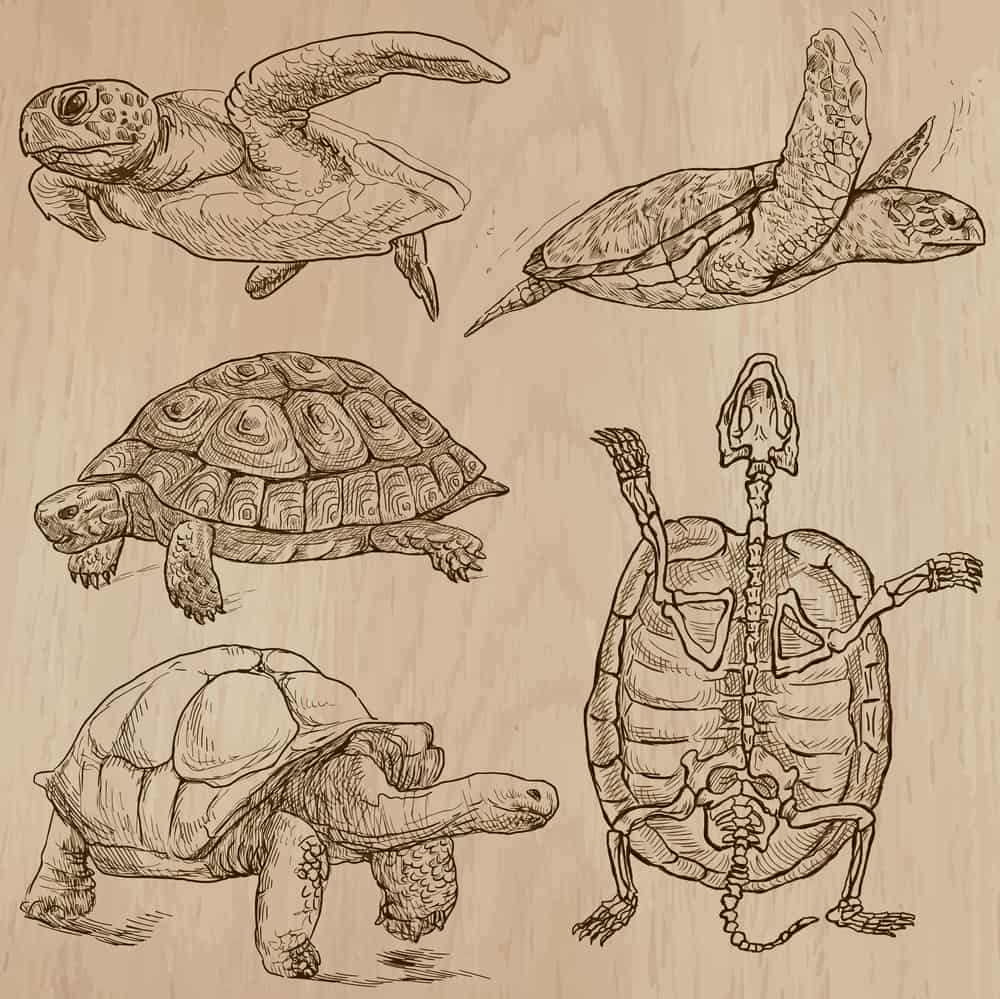This image appears to be a collection of intricately detailed pen-and-ink drawings of various turtles and tortoises on a light brown, wood-grained background. At the top right, a sea turtle is depicted mid-swim with its front flippers angled upwards, capturing a sense of movement underwater. To its left, another sea turtle extends its flippers out to either side, as if gracefully floating. In the middle, to the left, a box-type turtle (or terrapin) faces leftward, showcasing its distinctive shell patterns, visible legs, tail, and head with an open mouth. Below this turtle on the left, a large land tortoise is drawn in mid-step, characterized by its substantial feet, longer neck, and lighter-colored shell. To the right of this tortoise, a meticulous anatomical drawing reveals the skeleton and shell from the underside of a tortoise, displaying all the bones and skeletal structure. The professional-grade drawings, executed in dark ink, contrast sharply against the earthy, tan backdrop, emphasizing the diversity and anatomical intricacies of these reptiles.